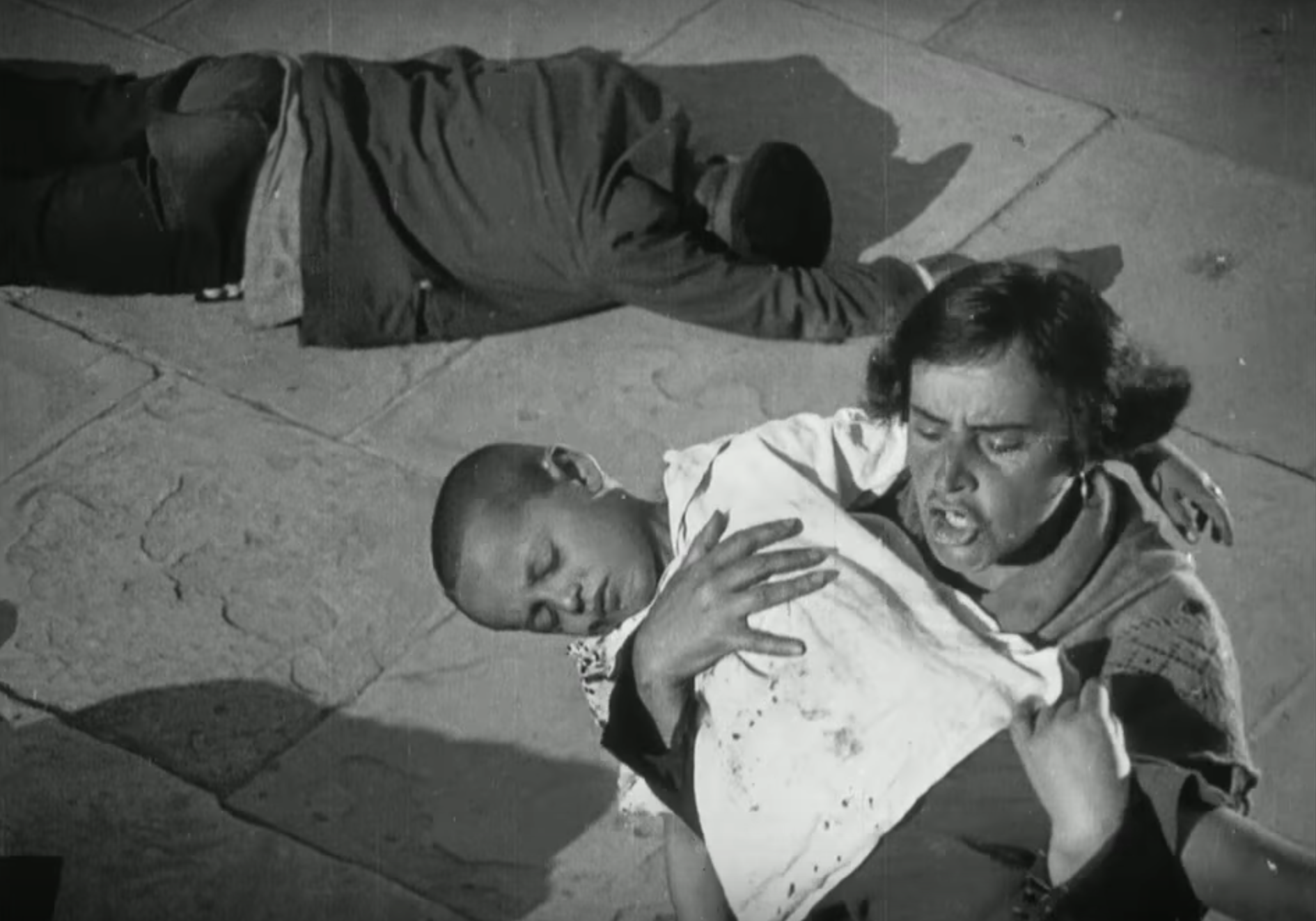This black-and-white image, possibly a screencap from a movie or a professional photograph, exudes a dramatic and distressing atmosphere. It captures three individuals situated on a cement block floor, clearly segmented into squares of concrete. 

In the background, dominating the top third of the image and extending across the left two-thirds, lies a man dressed in a long-sleeved black jacket over a lighter-colored shirt, paired with dark pants. His right arm is stretched above his head, and he appears to be face down, turning away from the camera. The shadows cast by the sun highlight his static form, suggesting he might be deceased.

In the foreground, situated in the bottom right corner, is a distraught woman with short, curly hair, her distressed expression accentuated by her closed eyes and open mouth, indicating a scream of agony. She cradles a young boy, about nine or ten years old, wearing a white shirt and dark pants. The boy’s eyes are closed, and his limp form suggests he might be deceased or gravely injured. The woman's appearance and emotional turmoil add a layer of profundity to this harrowing scene, conveying a narrative of recent tragedy and loss.